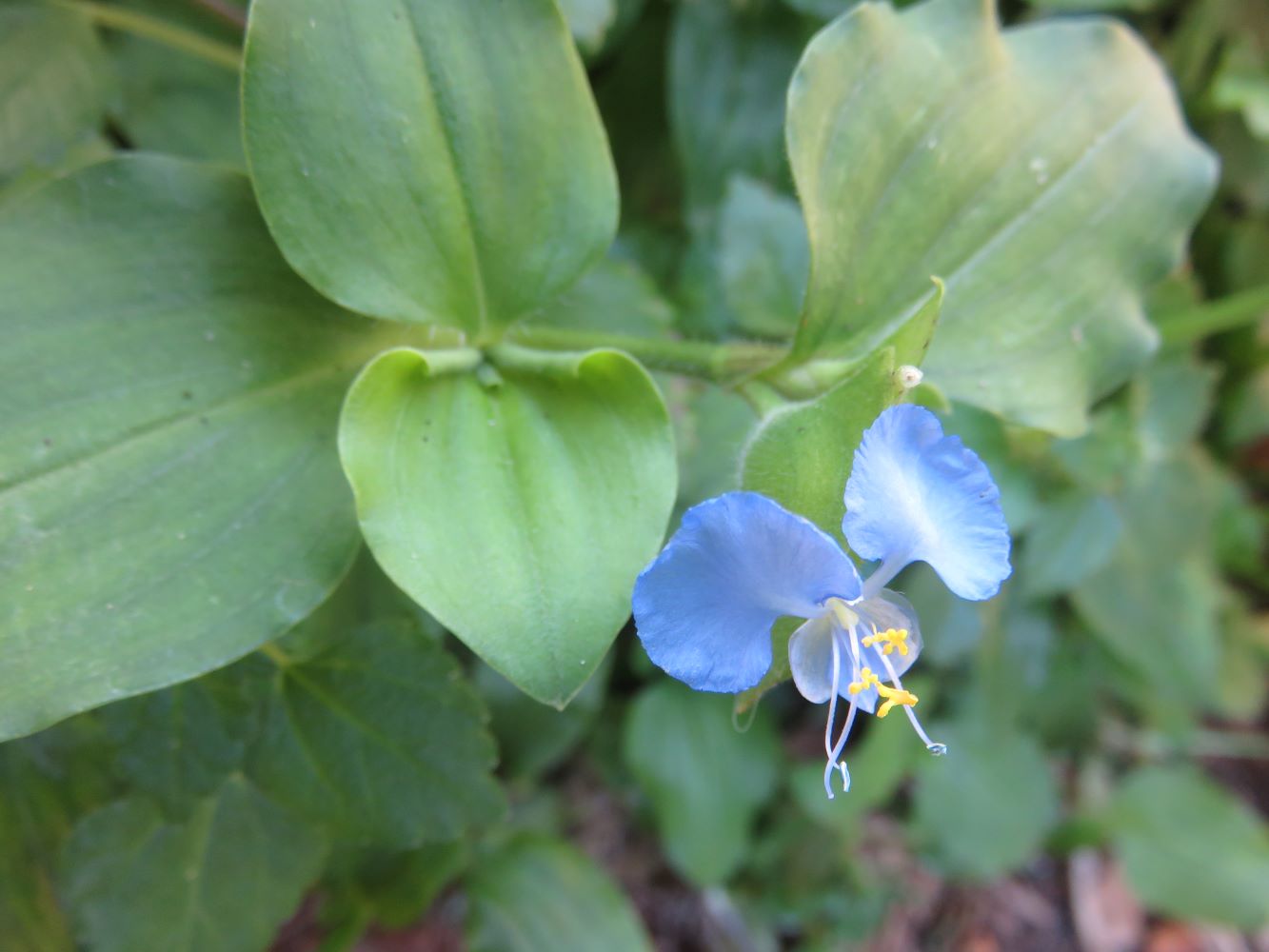This landscape-oriented photograph is a detailed close-up of a blue flower, prominently positioned just below and to the right of the center of the image, in the lower right quadrant. The flower features three delicate, heart-shaped petals with three slender, light blue stamens emerging from its center, each tipped with small yellow ends. This intricate blossom is attached to a plant adorned with green, heart-shaped leaves and a fuzzy stem.

Surrounding the blue flower, the immediate foliage is in sharp focus, particularly the green leaves in the upper left-hand quadrant of the image. One notable leaf to the left of the flower has its ends near the stem curled upwards. Towards the bottom left of the photograph, there's another type of leaf, smaller and serrated, offering a distinct texture compared to the larger, smoother ones. The background, populated with additional green leaves and some brown sticks and leaves, is softly out of focus, emphasizing the flower and its closest leaves as the primary subjects of the image.